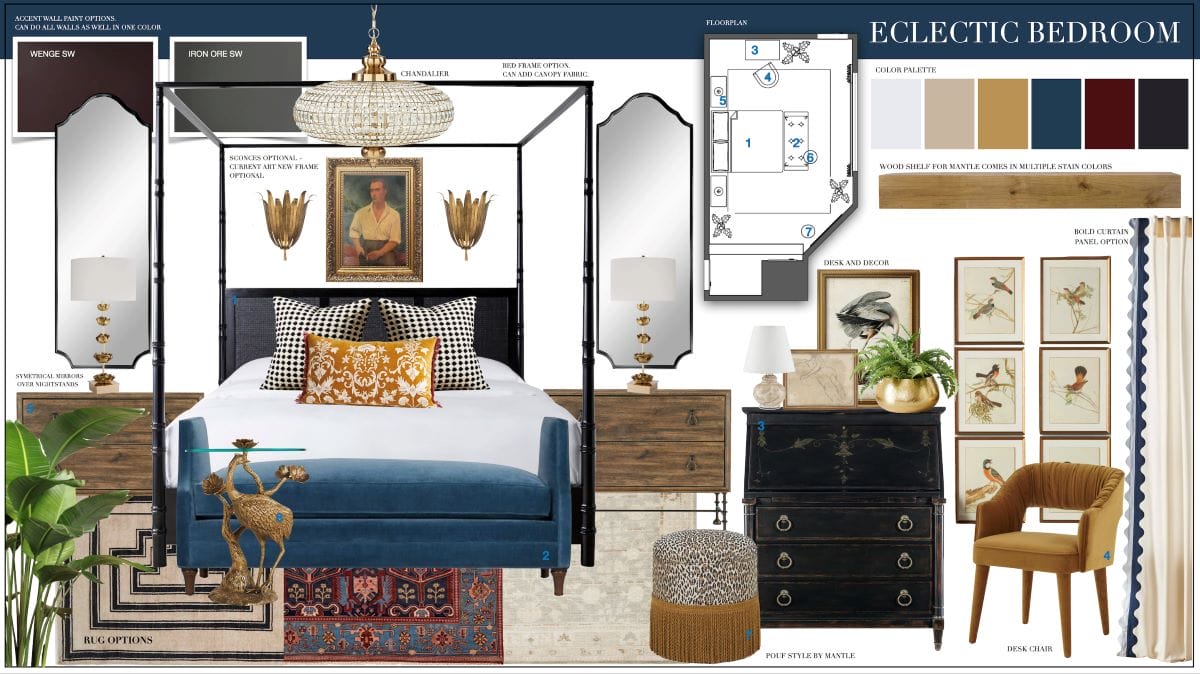The image showcases a meticulously curated mood board for an eclectic bedroom, presented in a collage style. At the top right is a header in a white, all-caps font against a dark blue background reading "ECLECTIC BEDROOM." The focal point is a four-poster bed adorned with checkered pillows, a gold throw pillow, and white sheets. A velour blue bench sits at its foot. Flanking the bed are two identical wooden two-drawer end tables, each with a lamp boasting a white shade. Close by are long mirrors accompanied by two color swatches in brown and gray. The mood board also includes a trio of rugs, suggesting a selection process for the room's final choice. Additional furnishings feature an animal print stool with tassels, a dresser embellished with artwork, and a yellow chair positioned near artistic renderings of birds. There is also a floor plan, mapping out the intended arrangement of these elements. The scheme is rounded out with various color swatches in shades like black, tan, brown, blue, light gray, maroon, beige, green, and light brown, reflecting the room's diverse palette. Scattered throughout are plants, an Asian rug, and a series of photographs intended for wall displays, all contributing to the room's eclectic style.